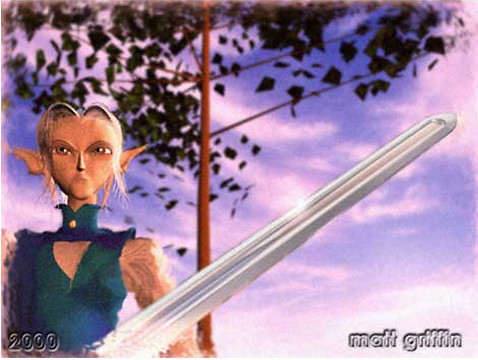The image is a detailed piece of digital artwork depicting an elf warrior set in a fantasy environment. The elf, positioned towards the bottom left of the frame, is facing the camera directly with an angry or stern expression on her face. She has pointy, long ears and white hair that barely touches her neck. Her attire includes a sleeveless, high-collared top in blue with some accounts suggesting it might be green and matching lower apparel, revealing her white skin tone and tattoos on her left arm. In her hands, she wields a long, white sword that extends from the bottom left towards the upper right of the image, featuring a fuller down its blade.

The background showcases a vibrant purple sky filled with clouds, adding depth to the scene. A thin tree with an orange-brown trunk and leaves is centrally located in the background, behind the elf. The bottom-right corner of the image is marked with the artist's name, "Matt Griffin," and the bottom-left corner features the year "2000" in a transparent color. There are additional bits of text in blue and white around these credits. The overall atmosphere suggests daylight, despite the purple hue of the sky.